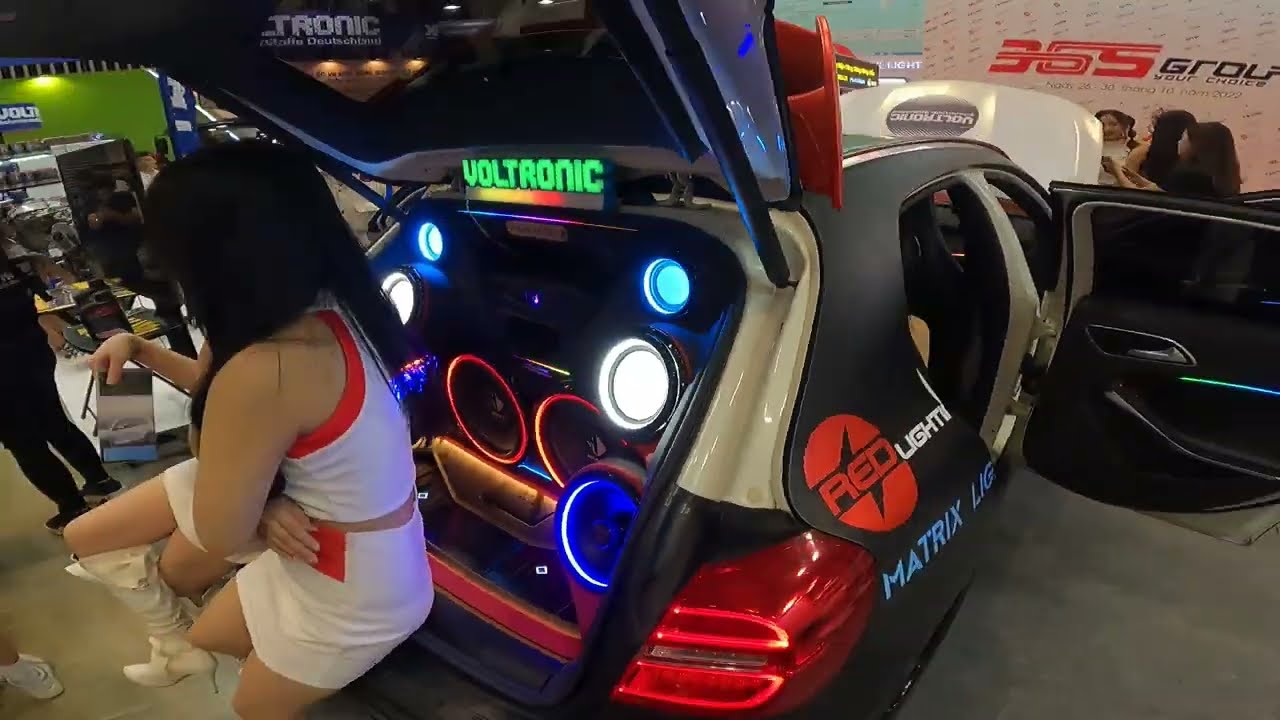The image captures a lively scene at a car show featuring a highly customized SUV emblazoned with the name "Voltronic" in green letters. The focal point of the photo is the spacious, open trunk filled with a dazzling array of brightly lit spotlights in various colors, including teal, white, red, and blue. Positioned in the trunk are two women dressed in coordinated white attire, including mini skirts, tank tops with red trim, and knee-high white boots. Both women appear to be engaging with someone nearby, though their faces are obscured, with one woman's black hair turned away from the camera.

The SUV, which also has its doors and hood wide open, showcases additional text on its body that reads "Red Light Matrix Light." To the right of the vehicle, an open door further highlights the detailed customization. In the background, a banner with the phrase "365 Grow" or "3 6 S Group, Your Choice" is partially visible, adding to the sense that this event is a bustling conference or exhibition. Around the car, several people are gathered, including three more women near the front of the vehicle, one of whom sports bubble ponytails and a white shirt, while another wears a black top with long brown hair. The overall atmosphere is vibrant and crowded, indicative of a major promotional event.